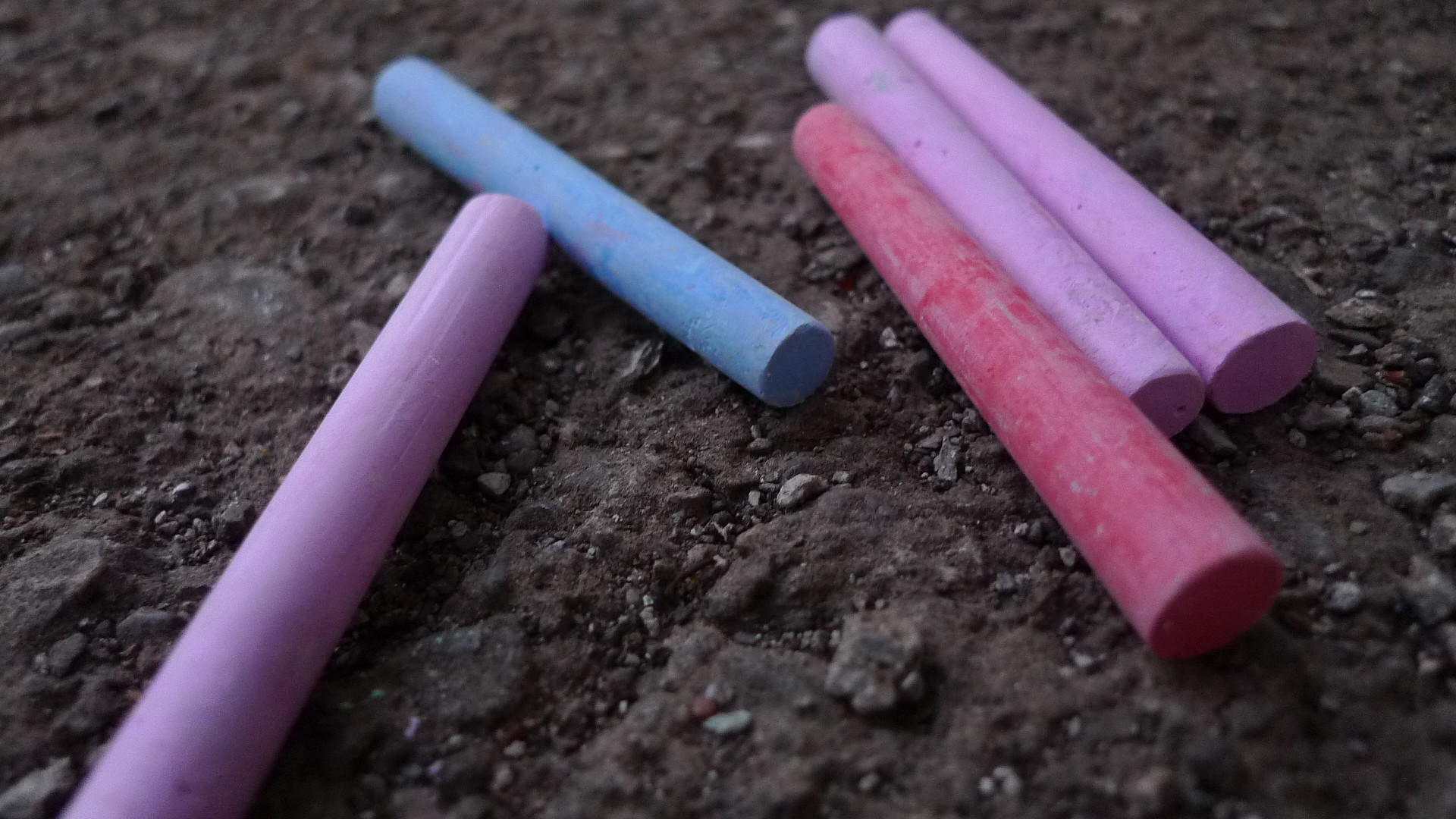This is a close-up photograph of five brand new sticks of chalk laying on a textured, brown dirt and rocky ground. The chalk pieces are arranged next to each other, with two being purple, one blue, one red, and one lavender. The surface of the red chalk has a notable white chalky residue. The image sharply focuses on the chalks, highlighting their vivid colors and pristine condition, while the surrounding ground appears blurred, drawing attention to the fresh, unused sticks as the main focal point.